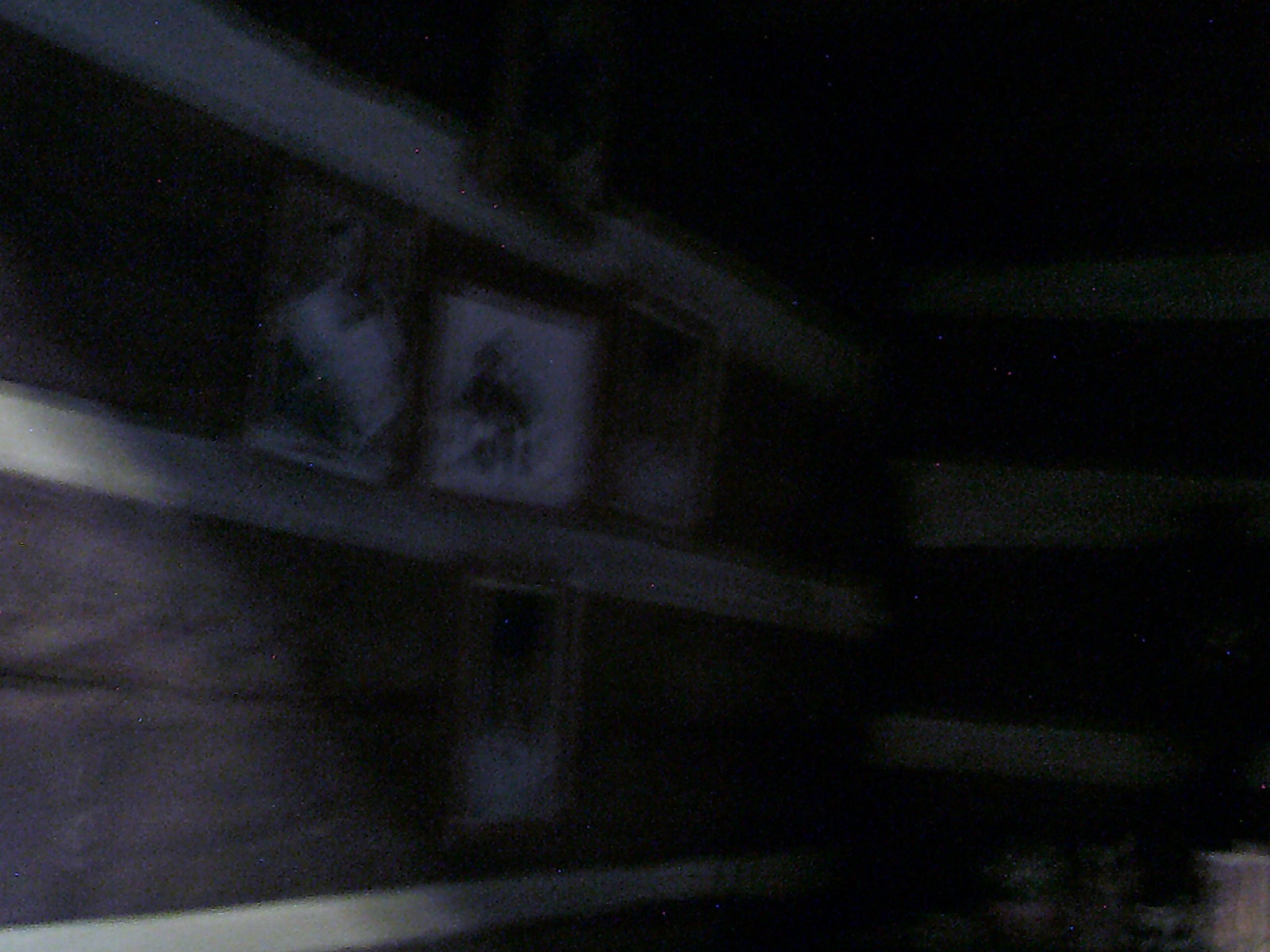This is a photo of a dimly-lit and blurry corner of a room, likely inside a building or home. The image is generally dark, with the walls and objects within appearing indistinct due to the graininess. Two walls are visible in the shot. 

On the left wall, five pictures or paintings are arranged in a cross pattern: one at the top, three in the middle, and one at the bottom. The images are possibly of people, but the blurriness makes it difficult to be certain. This wall features three horizontal white trims positioned at the top, middle, and bottom sections. 

To the right, there is another wall that also has three rows of white trim, creating a grid-like appearance with square sections. Near the bottom right of the image, some white objects, potentially candles or cups, are barely visible. Additionally, there seems to be a faint light source on the left-hand side of the wall, contributing to the overall dark ambiance of the photograph.